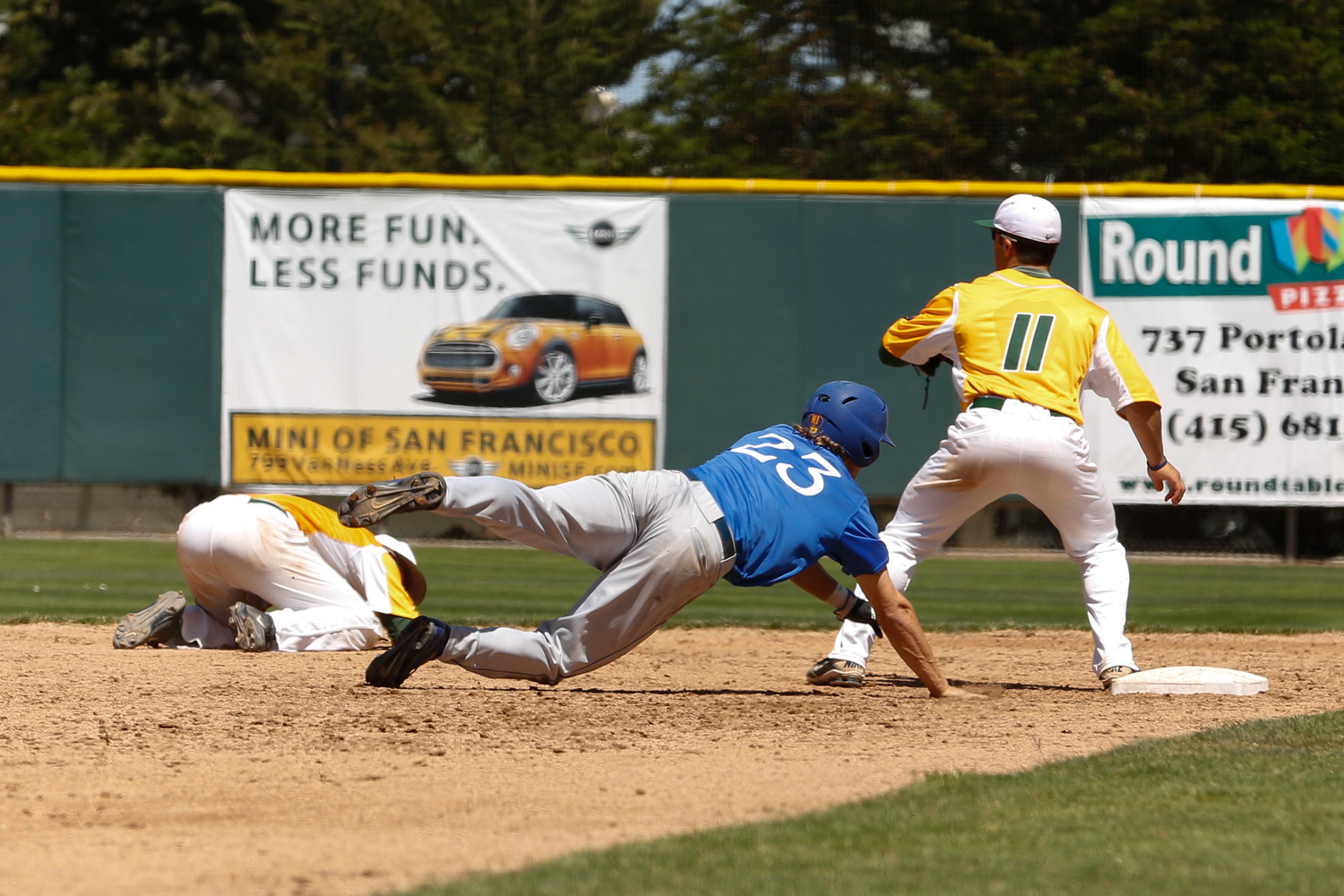The image captures a lively moment during a daytime baseball game. In the foreground, a player from the blue team, wearing a blue helmet, a blue shirt with the number 23 in white, and gray pants, is sliding aggressively into a base. The base is manned by a player from the yellow team, who is wearing a yellow shirt with a green number 11, white pants, and a white baseball hat with a green bill. This player is bracing to catch the ball to tag the sliding runner. To their right, another player in a yellow uniform with white pants is on his knees with hands on the ground, seemingly in the midst of an attempt to assist or field the ball. The field itself is dusty, with a patch of dull green grass that looks under-watered surrounding it. In the background, the outfield fence is adorned with advertisements. The more prominent ad reads "More Fun, Less Funds, Mini of San Francisco, 799 Valmes Avenue," featuring a small car. Another ad, partially out of view, mentions "Round Pizza" with the rest of the details obscured. The scene is framed by a yellow line running atop the outfield fence, encapsulating a quintessential moment in amateur baseball.